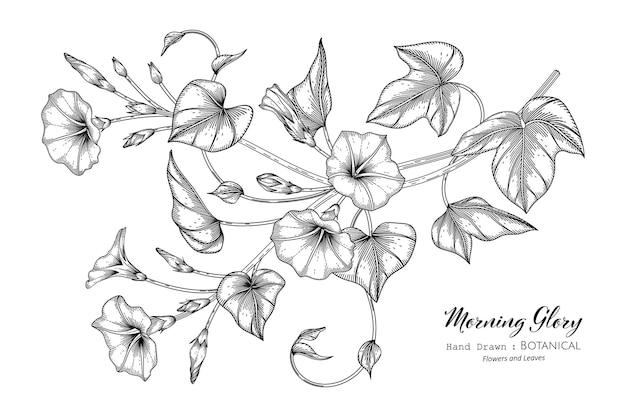In this black and white hand-drawn botanical illustration, we see a detailed depiction of Morning Glory flowers. The main stem, which begins in the top right corner and extends down to the bottom left, features branches that split off towards the top left and bottom left. This main stem is adorned with four large leaves, extending in various directions, some featuring three distinct lobes.

Two prominent trumpet-shaped, or bell-shaped, flowers are situated on the main branch, pointing in opposite directions. Additionally, the illustration includes several buds that have yet to bloom, emphasizing the plant's stages of growth. There are curled vines wrapping around the branches, adding a touch of natural intricacy. The entire plant appears to be suspended in space, not rooted in any particular ground.

In the lower right corner of the image, the text "Morning Glory" is elegantly scripted in cursive, with the words "Hand Drawn, Botanical, Flowers, and Leaves" printed below it in a simpler font. The meticulous shading and detailed line work bring a lifelike quality to this impressive sketch, capturing the essence of the Morning Glory plant in beautiful monochrome.